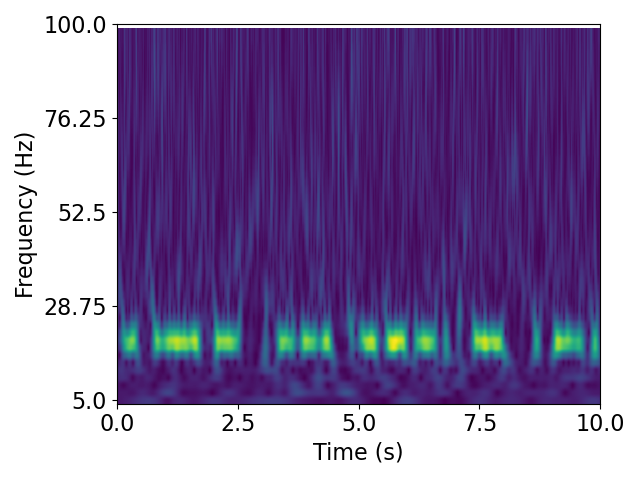The image depicts a detailed time-frequency graph with time measured in seconds along the x-axis (ranging from 0 to 10 seconds) and frequency in hertz along the y-axis (ranging from 5 to 100 Hz with marked intervals at 28.75, 52.5, and 76.25 Hz). The graph is primarily dark blue, indicating the absence or low intensity of frequencies over most of the period. However, notable signatures in green appear around the 20 Hz frequency, showing intermittent activity with small gaps over the 10-second span. The overall resemblance of the graph to an oscilloscope suggests complex data representation, challenging to interpret at first glance.